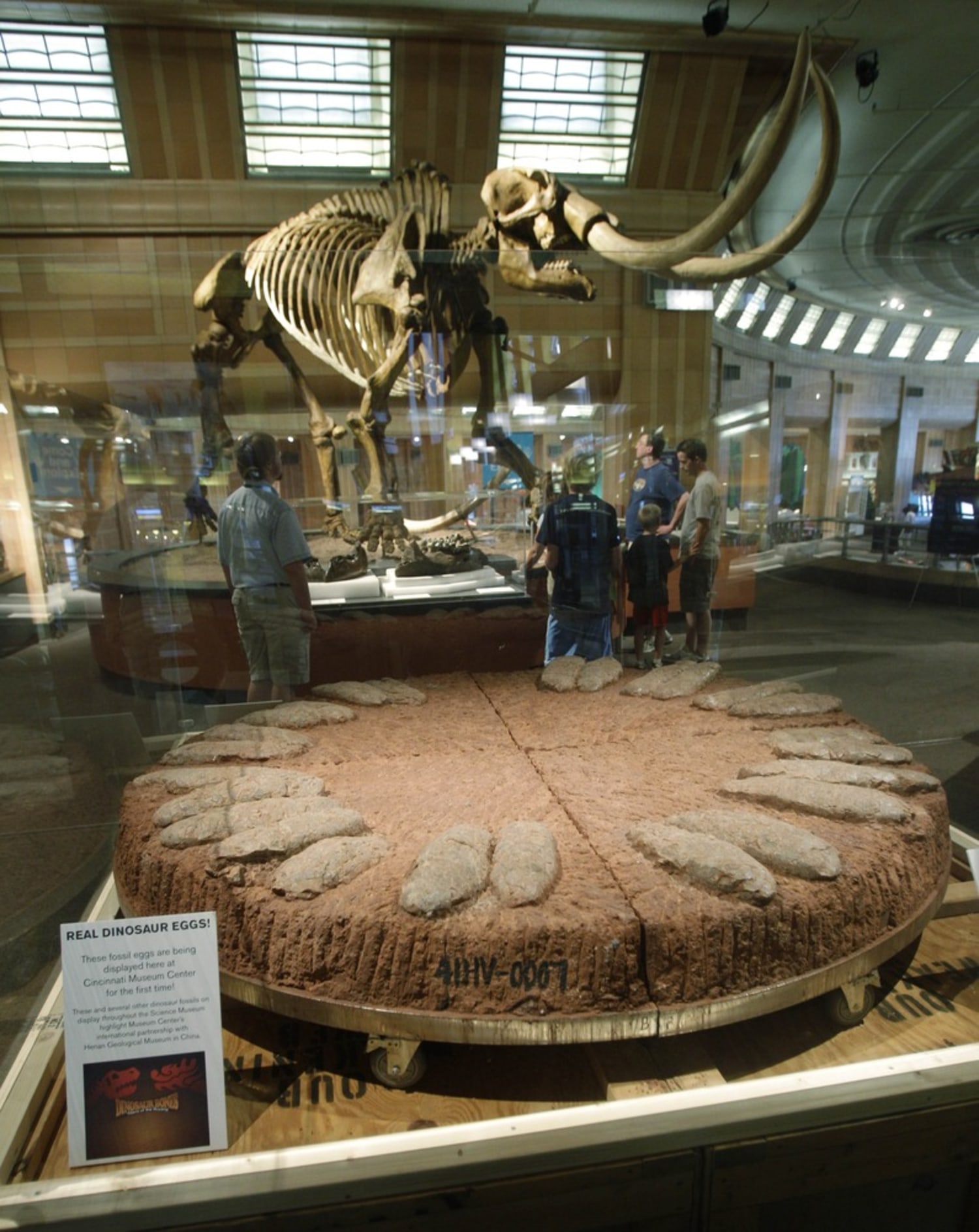This photograph showcases an engaging exhibit at the Cincinnati Museum Center. In the foreground, prominently displayed in a square glass case, are real fossilized dinosaur eggs. These eggs, which are oval-shaped and gray, rest on a hardened mound of sediment, evoking the earth they were discovered in. The sign beside this display confirms their authenticity. In the background, visitors can be seen marveling at an impressive woolly mammoth skeleton. This colossal prehistoric creature, with its enormous tusks, stands tall, nearly reaching the ceiling, and commands the attention of five onlookers, including adults and children. The museum’s grand rotunda and high windows, which bathe the scene in natural light, add to the grandeur of the exhibit. The setting features a light brown stone facade and a concrete museum floor, enhancing the historic and educational ambiance.